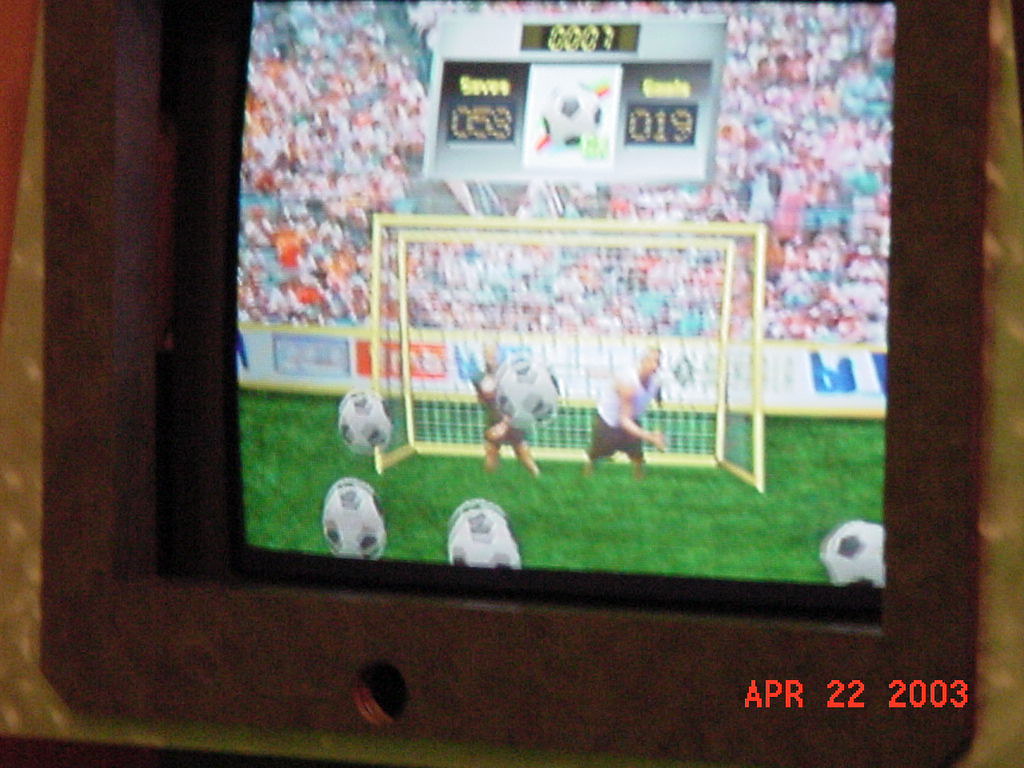The image depicts a slightly blurry close-up of an old, wooden-framed television screen, dated April 22, 2003. The TV is showing a lush green soccer field with a packed stadium full of indistinct, animated spectators wearing various colors such as greens, oranges, and whites. The main focus is a yellow goal where two Caucasian men, potentially the same person in different positions, are visible in front of the net. One of the men appears to be performing a follow-through motion of a throw, with his blonde hair and white muscle shirt standing out, while the other man's torso is partially obscured by a flying soccer ball. In total, there are five soccer balls visible on the field; four are aimed at the goal, while the fifth is off to the right.

Above the goal, a scoreboard indicates the game details, showing seven seconds left. The left side displays a score of 53, possibly indicating saves, while the right side shows 19, potentially goals, with a soccer ball logo positioned between the scores. The bottom right corner of the TV screen prominently features the date stamp. The advertisements and wall graphics separating the field from the spectators are blurred, making specifics indiscernible. Overall, the picture captures the dynamic essence of the soccer game within the aesthetic of an old tube television, set within a dark brown wooden frame with rounded corners.